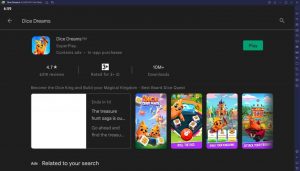The image appears to be a low-resolution screenshot of a dark-themed Google Play Store listing for a mobile app called "Dice Creatures." The primary icon is of an orange character set against a blue background. Beneath this icon, there's a line of text indicating the app is available on Google Play, along with a green button labeled "Play." The app has a rating of "4.7 stars" and boasts "10 million+ downloads." To the right, four smaller screenshots showcase gameplay elements: the first image features the orange character with a companion, the second shows him interacting with dice, the third places him in front of a castle, and the fourth displays another character with clouds and a castle in the background. The text "Rated for 3+" indicates the app's age suitability. At the bottom of the image, there is a section titled "Ads related to your search."